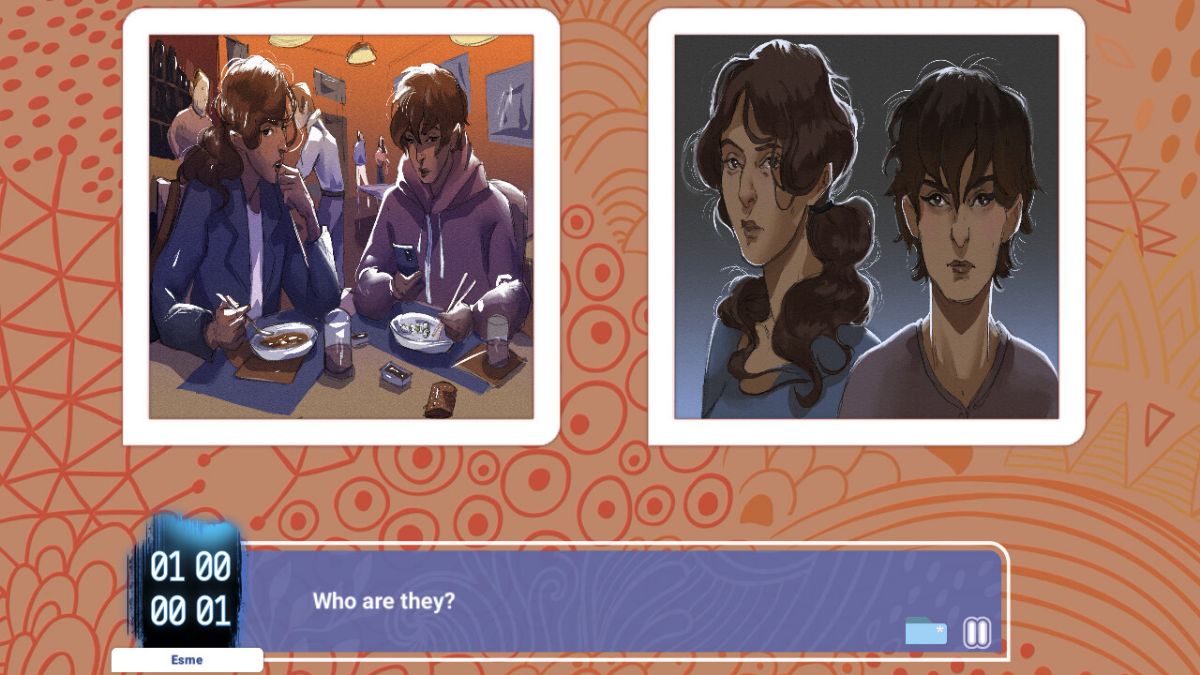Landscape-oriented anime screenshot featuring a dual-image collage with intricate background

This landscape-oriented image, roughly twice as wide as it is tall, presents a vividly detailed anime scene. The background is bathed in a pink hue, interspersed with myriad lines and patterns forming an enigmatic design, accentuated by yellow lines and circular motifs.

In the upper half of the image, two photos are highlighted, each encompassed by a clean white frame. The first photo on the left depicts a cozy restaurant or diner setting. Here, a woman with long brown hair, wearing a blue jacket, is engaged in eating from a bowl. Beside her, a man in a light purple hooded sweatshirt holds a cell phone in one hand while skillfully using chopsticks with the other.

The second photo, situated to the right, features the same duo but in a starkly different ambiance. With a grey background, both characters stand side by side, now dressed in blue and purple shirts, respectively. Their expressions are notably serious, offering a sharp contrast to the more casual, relaxed demeanor in the first image.

Along the bottom of the scene, a white text bubble on a blue background displays text in white font. To the left of this bubble, a box shows the numbers "0100" and "0001" stacked vertically. Adjacent to this box on the right, a pause icon and another unidentified element suggest this image is taken from a video, likely from an anime or animated series.